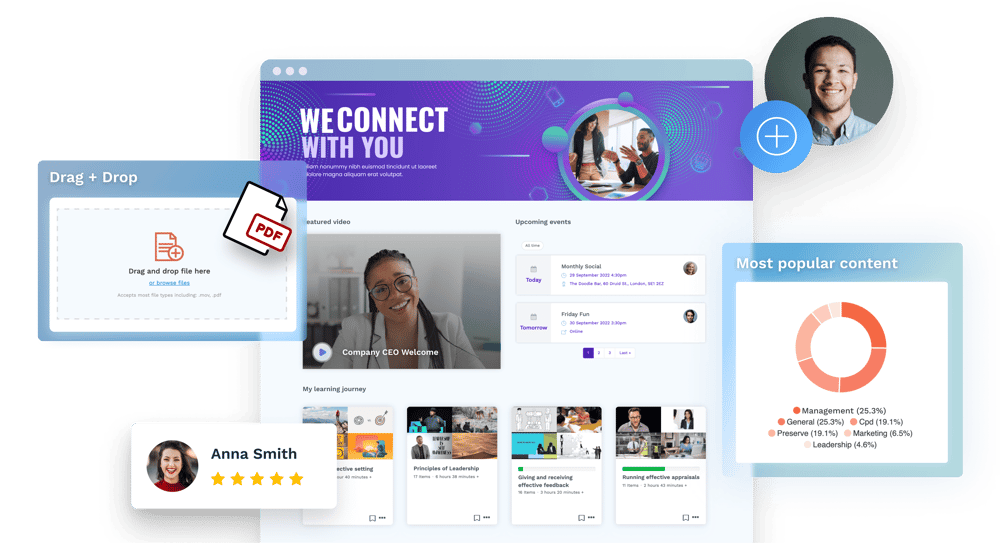This image is a screenshot of a website with a busy and colorful layout. Dominating the center is a large square section, extensively overlaid by three pop-up boxes. The primary color scheme features white, purple, light blue, yellow, and accents of orange.

At the forefront, a prominent purple banner announces, "We connect with you." Below this banner, a circular photograph showcases two people, and beneath this, a video of a smiling woman with her head tilted to the left is displayed. Further down, there are four distinct sections, each containing four photographs and accompanying text descriptions.

To the left side, partially overlapping the central square, there's a drag-and-drop box designated for PDF files. Below this box, the text "Anna Smith" is displayed along with five yellow stars indicating a rating, and her profile picture is positioned to the left of her name.

In the top right corner, an addition button in a blue circle features a man's profile picture. Directly beneath this, another square pop-up box labeled "Most popular content" contains an orange and white grid.

A section below the purple banner is titled "Upcoming Events," listing two events underneath it.

The image has a white background with no discernible border, contributing to its clean yet dynamic appearance.